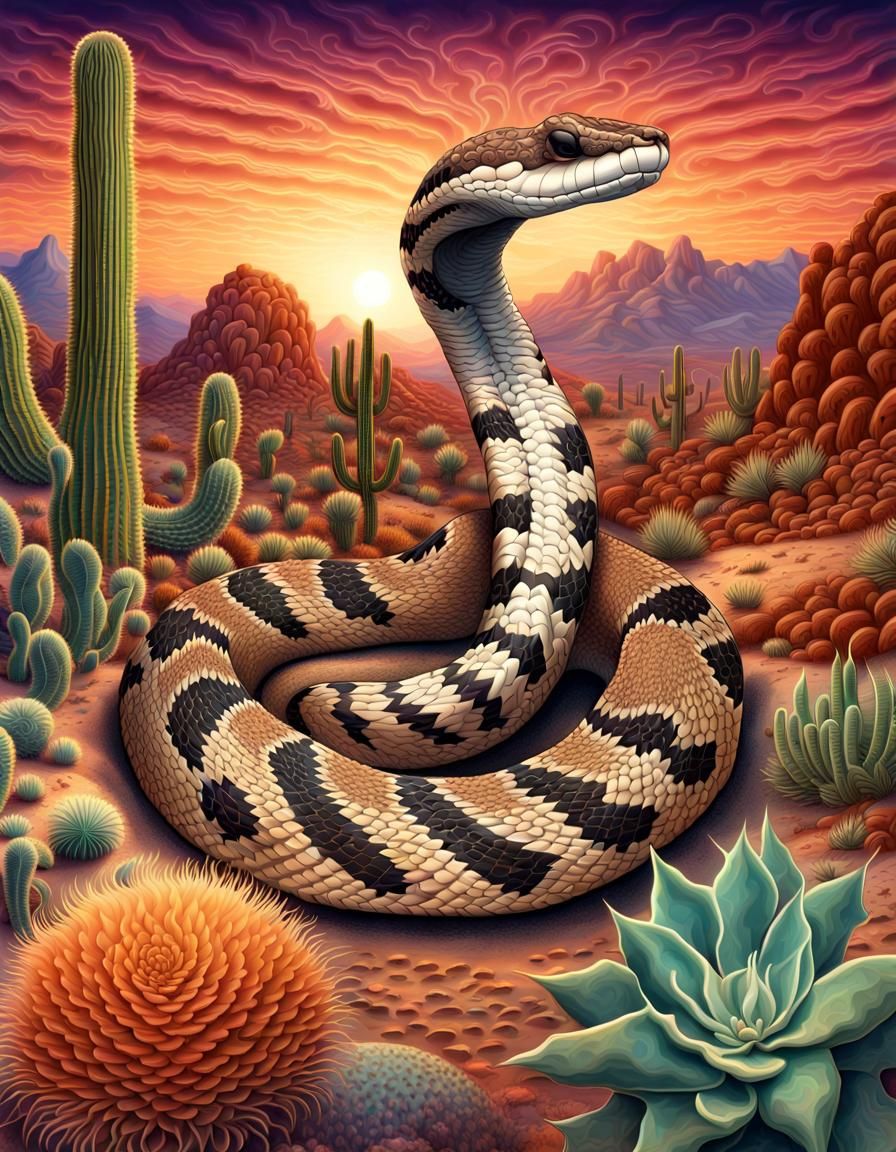The image is a highly detailed, vibrant illustration, potentially AI-generated or a painting, showcasing a colossal snake as the central focal point. The snake, depicted in a close-up view, is coiled with its neck and head raised, giving the impression that it is observing something. Its scales are meticulously illustrated, featuring a striking pattern of brown with black stripes, and its expressive brown eyes are open. Surrounding the snake is a desert landscape populated with a diverse array of cacti, including traditional, flower-like, bulbous, and trident-shaped varieties, each rendered in different shades of green and orange, complete with sharp, needle-like prongs. In the background, rounded, reddish-brown rocky hills and mountains are visible, made up of spherical stones stacked atop each other. The sky is awash with vibrant hues of orange, yellow, and pink, suggesting either a sunrise or sunset, and is marked with wavy yellow lines, enhancing the modern and surreal aesthetic of the scene.